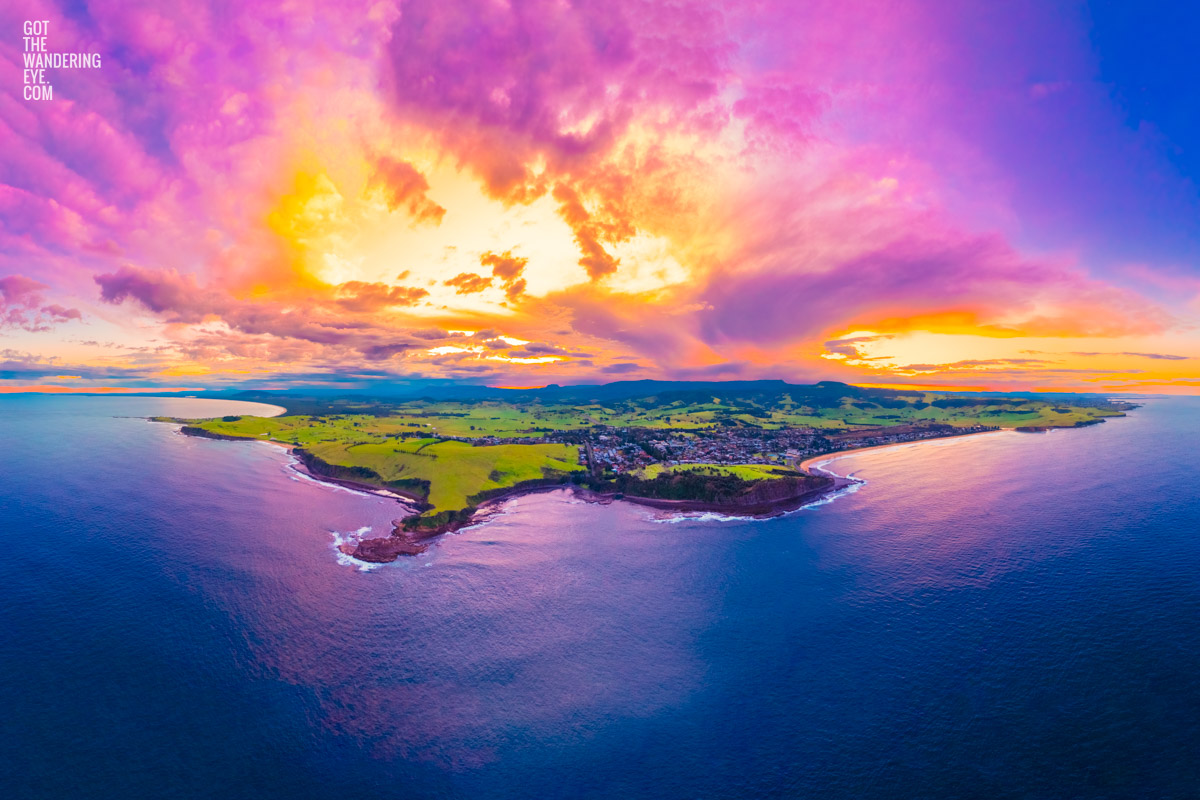The image depicts a breathtaking and vibrant outdoor scene dominated by a vast expanse of deep blue water, gradually lightening as it approaches a distant, grassy peninsula. The sky is an astonishing mix of colors, including shades of yellow, orange, pink, purple, fuchsia, magenta, and both light and dark blue. A hint of an orange-colored cloud with magenta hues adds depth to the vivid sky. The horizon features a light landmass, with the grassy peninsula standing out in light green. In this scenic view, faint outlines of towns can be seen along the coastline, though details remain obscured by the colorful atmosphere. The bottom left-hand corner of the image discreetly features the text, “got the wandering eye.com,” adding a subtle branded touch to this mesmerizing landscape.